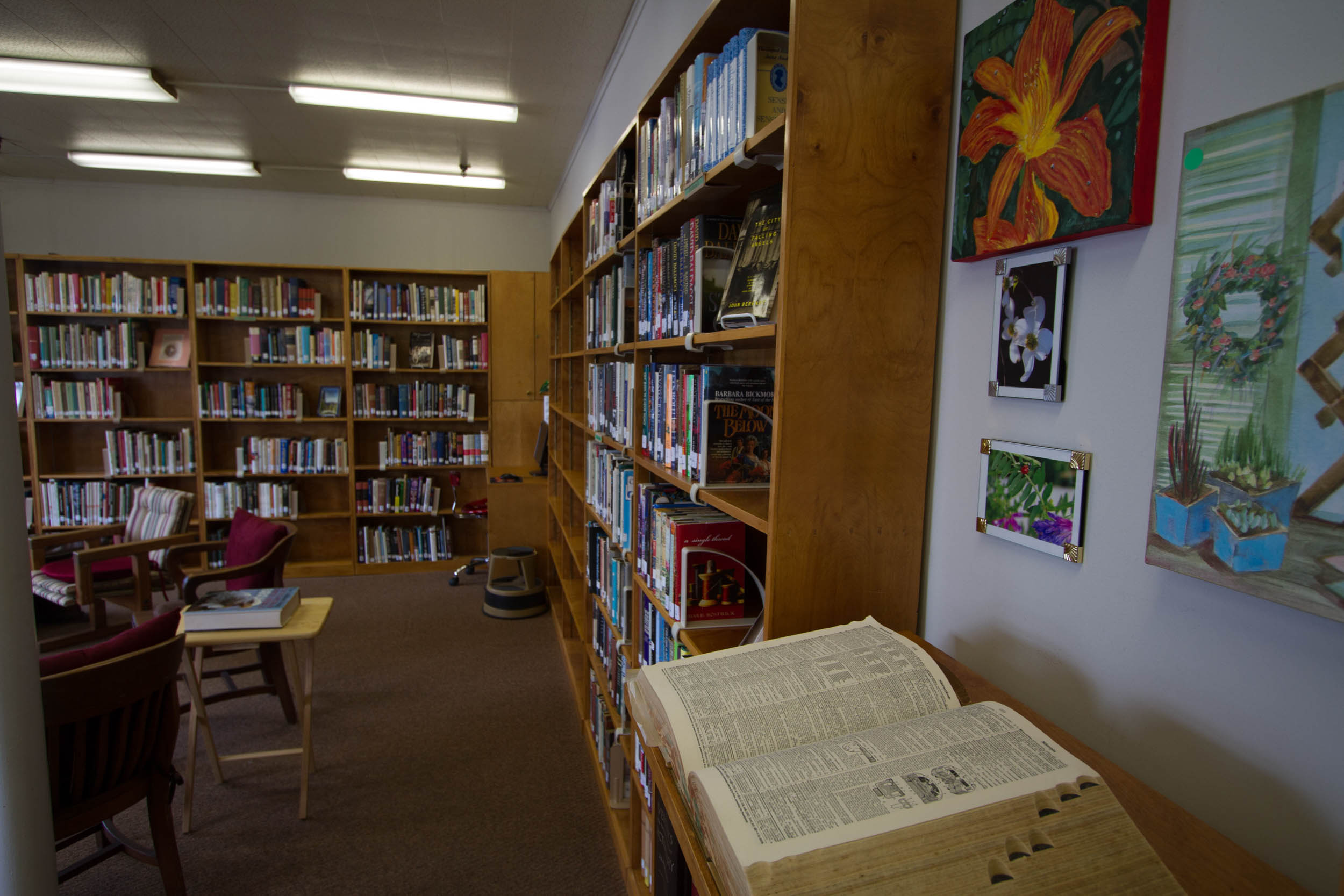This detailed image captures an inviting library in a landscape orientation, filled with various elements of academic and leisure character. Dominating the right side and the back wall, there are medium-toned oak bookshelves, each featuring six shelves sparsely populated with neatly arranged books. Some of these books are displayed front cover forward among the side-spine-facing ones, all held in place by semi-circular book stops. In the back right corner, a metallic footstool typical of retail shops stands ready for use, boasting three rungs with a black trim and tread atop its brown carpeted setting.

Further enriching the right side, a large, open book with yellowed pages rests on a brown cabinet, hinting at the allure of a dictionary or an encyclopedia, characterized by thumb labeling for easy navigation. Above this cabinet, the wall displays four slightly cut-off paintings, showcasing vibrant floral and garden themes.

To the left, partially visible around a corner, is a cozy seating area featuring an array of comfortable chairs with wooden arms. These chairs, some adorned with red and striped cushions, form a semi-circle arrangement, inviting quiet study or interaction. A TV dinner-style collapsible table in light-colored beech wood sits near the frontmost chair, bearing a large book that nearly covers the table's surface.

The overhead white strip lights cast a clear glow over the room, while the ceiling features evenly spaced rows extending from left to right, enhancing the well-lit, welcoming atmosphere of this academic haven. The image encapsulates the serene but bustling environment typical of a well-loved library space.